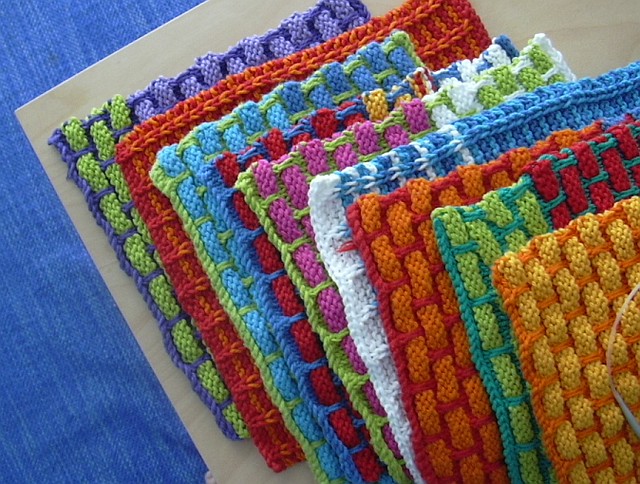This photograph showcases approximately eight to ten small, hand-woven quilt squares, each uniquely designed with an intricate blend of colors. The quilts are stacked in a way that allows a glimpse of each vibrant pattern. Notably, the bottom-most square features light green and purple, accented with dark blue threading. Moving up, there's a red and orange square, followed by a light blue and green one. Another square consists of a darker blue intertwined with red, while one above it mixes purple-pink and green. There's also a notable combination of white and blue, and another with striking lime green and purple hues. Additional squares include patterns of orange and yellow, lime green with light yellow, and one with a rich red color mixed with lighter orange.

These carefully crafted quilts rest on a wooden surface, likely part of a table, which is adorned with what appears to be a blue denim-like material reminiscent of a pair of blue jeans. This layered presentation not only highlights the individual color combinations and designing techniques—such as knitting, crocheting, and sewing—but also provides a textured, rustic background that complements the artisanal quality of the quilts.